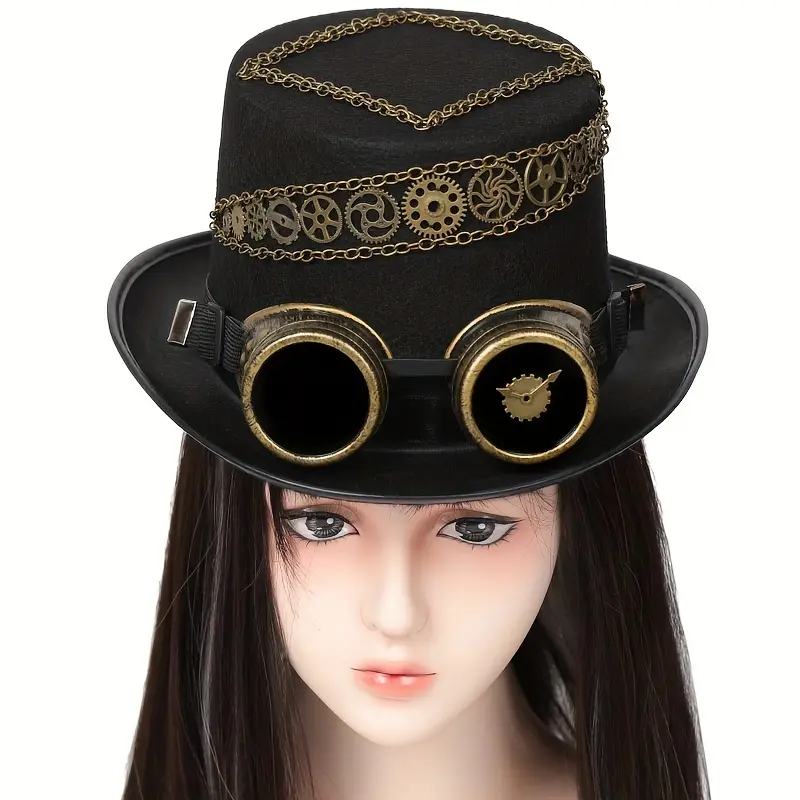This image depicts a female mannequin adorned with a steampunk-themed ensemble. She wears a black wig with a prominent blonde streak, complementing her detailed and elaborate top hat. The tall black hat is adorned with various metal decorations, including multiple gears that come in different shapes like circles and spiral patterns, giving it an intricate appearance. Attached to the hat are brass steampunk goggles, with one eyepiece featuring an elaborate gear mechanism with clock hands, adding to the vintage industrial aesthetic. Chains interlink the gears around the hat, forming a decorative outline above the brim. The hat also features a small belt buckle on the inside of the brim, further enhancing its detailed design. The mannequin stands against a white background, emphasizing the striking details of her steampunk attire.